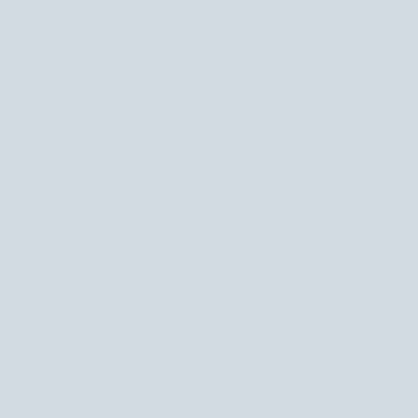The image features a perfectly square, medium-sized box with a light gray background. The box's dimensions appear to be approximately two inches in both width and length. The light gray background is uniform, with no pixelation, and the box's edges are sharp and even on all four sides. Surrounding the gray square is a very thin, almost imperceptible blue border, adding a subtle accent to its appearance. The overall simplicity and neutrality of the gray shade suggest that this might be intended as a placeholder or background for a company icon or web element. The white space around the gray square is likely the screen or document background and not part of the image itself. If text were to be added to this light gray background, it would likely be in a contrasting color, such as black or white, to ensure readability.